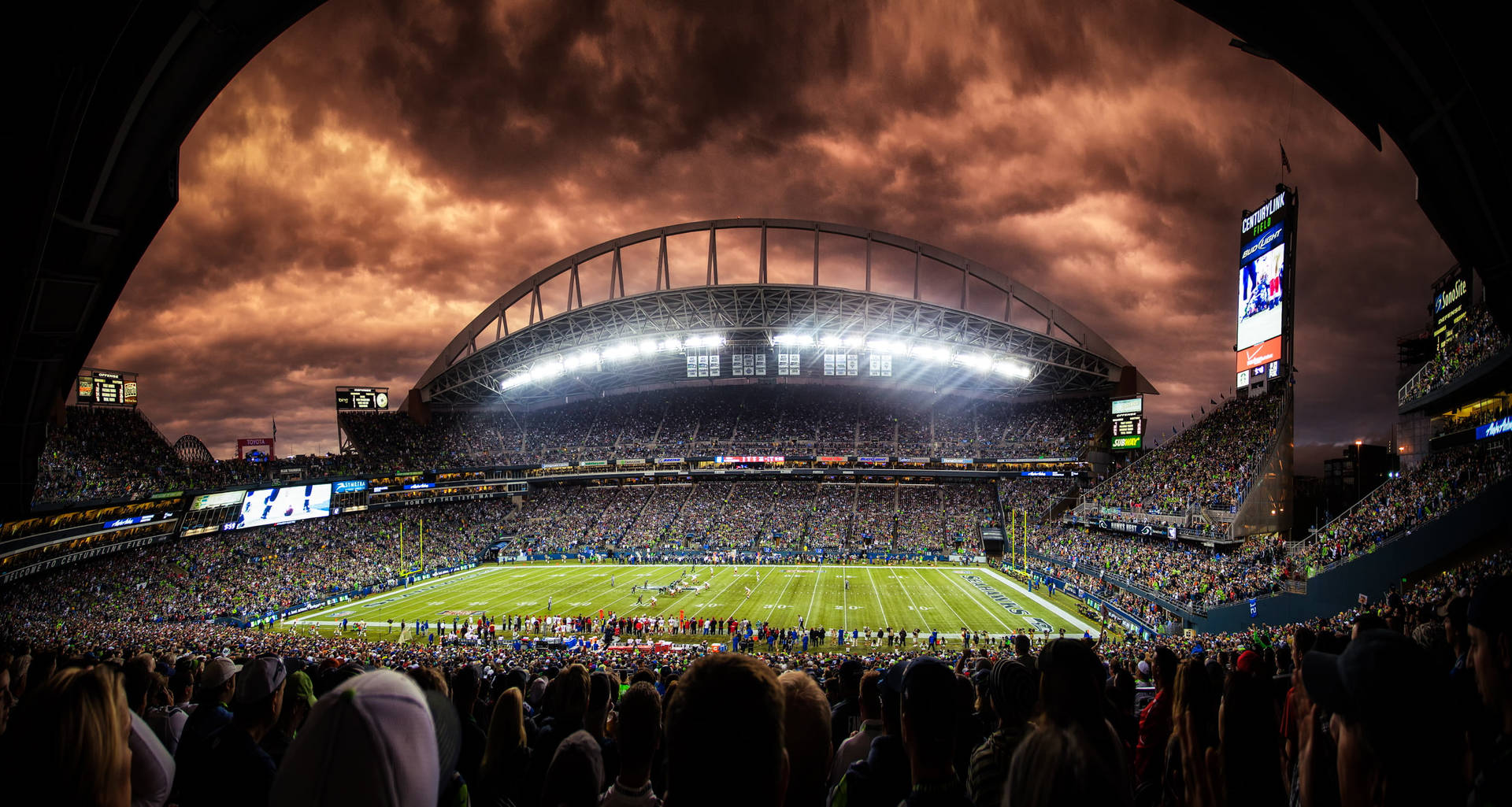A highly detailed photograph captures the grandeur of an American football game played in a large, packed stadium. Taken from the vantage point of the 20-yard line in the stands, the image frames the entire stadium, which includes both end zones and the crowded seating areas. The field is a lush, vibrant green, and players are assembled near the 50-yard line. The stadium boasts a prominent arch structure directly opposite the camera, illuminated by bright white lights. To the right, a large scoreboard is partially visible. Above, a dramatic sky unfolds, swirling with heavy clouds tinged in golden brown hues. The sky's texture and color hint at a recent sunset, adding an almost tie-dye effect to the stormy atmosphere. Despite the crowded stands and the unclear team identities, the image balances the action on the field with the imposing architectural and atmospheric elements, creating a vivid portrayal of a spirited football game amidst a grand and stormy setting.